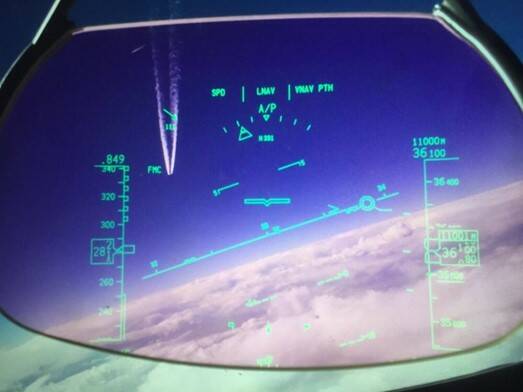This image captures the cockpit view from an aircraft, presenting a detailed and layered scene. Through a rounded glass screen, the expansive blue sky transitions from bright to dark hues, dotted with white contrails from another plane flying overhead. Below, a layer of fluffy white clouds stretches out under the horizon. On the interior screen, a diagonal line representing the horizon intersects the display, which is filled with green digital text and numbers providing aircraft data. On the left side, it reads "849" along with a number chart, while on the right, figures like "11,000 M" and "36 100" are visible. Additional markers such as "SPD," "LMAV," "PTH," and "A/P" are scattered across the screen, contributing to the detailed navigational information. The scene is framed by a black, oval-shaped border, encapsulating the high-altitude aviator's perspective.